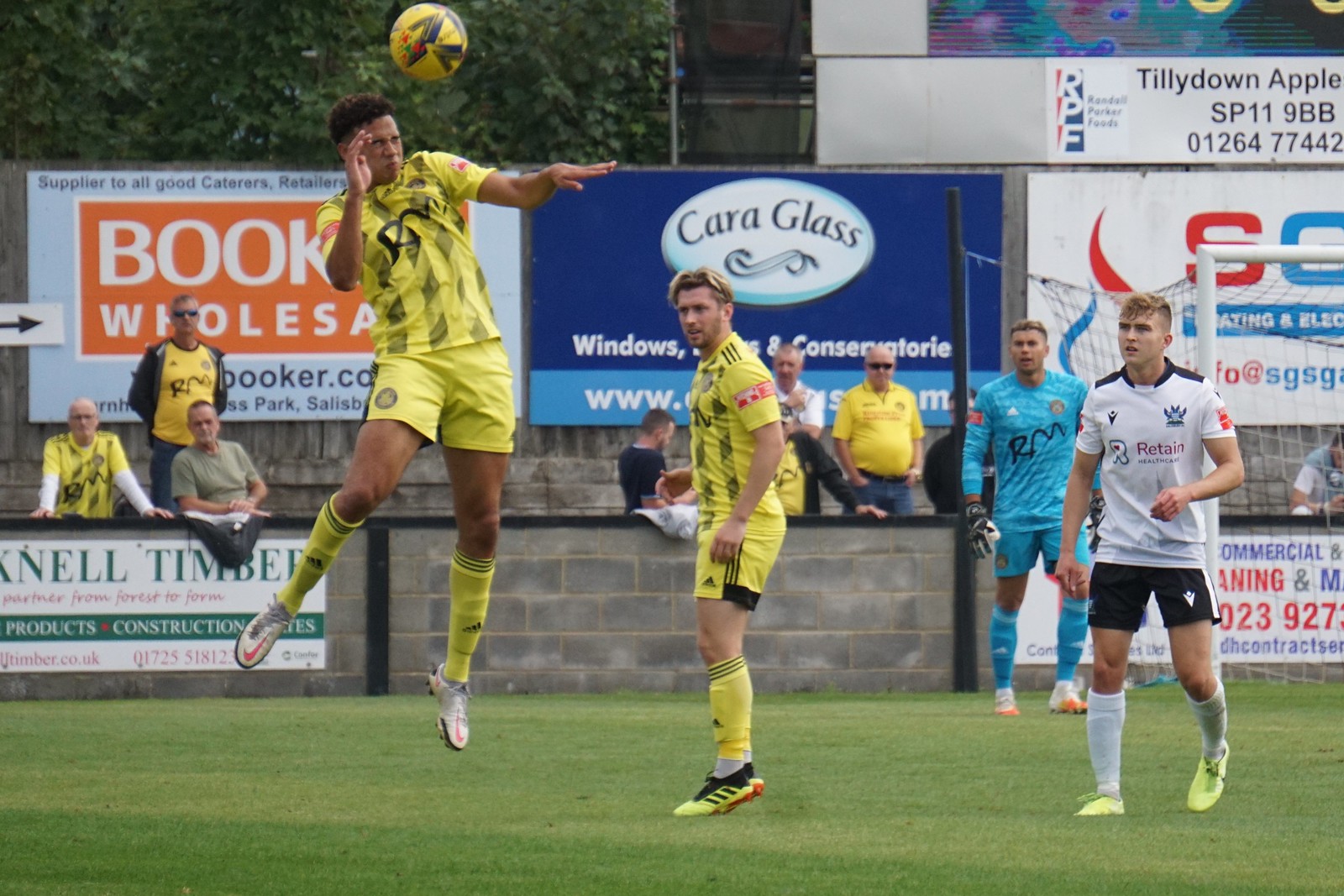In this vibrant, recent photograph from a professional soccer match, a player in mid-air is flinching as a yellow and black soccer ball slams into his face. Surrounding him, on a lush green soccer field, are other players in striking black and yellow jerseys, with one wearing all blue—likely the goalie. Another player in white and black stands off to the right. Behind this lively action, a cinder block wall separates a modest crowd from the field, adorned by numerous advertisements for services like book wholesales, car glass, and heating and cooling. Though a small audience watches from behind the wall, the intensity and professional demeanor of the game are palpable, with the home team's colors dominating both the field and the stands.